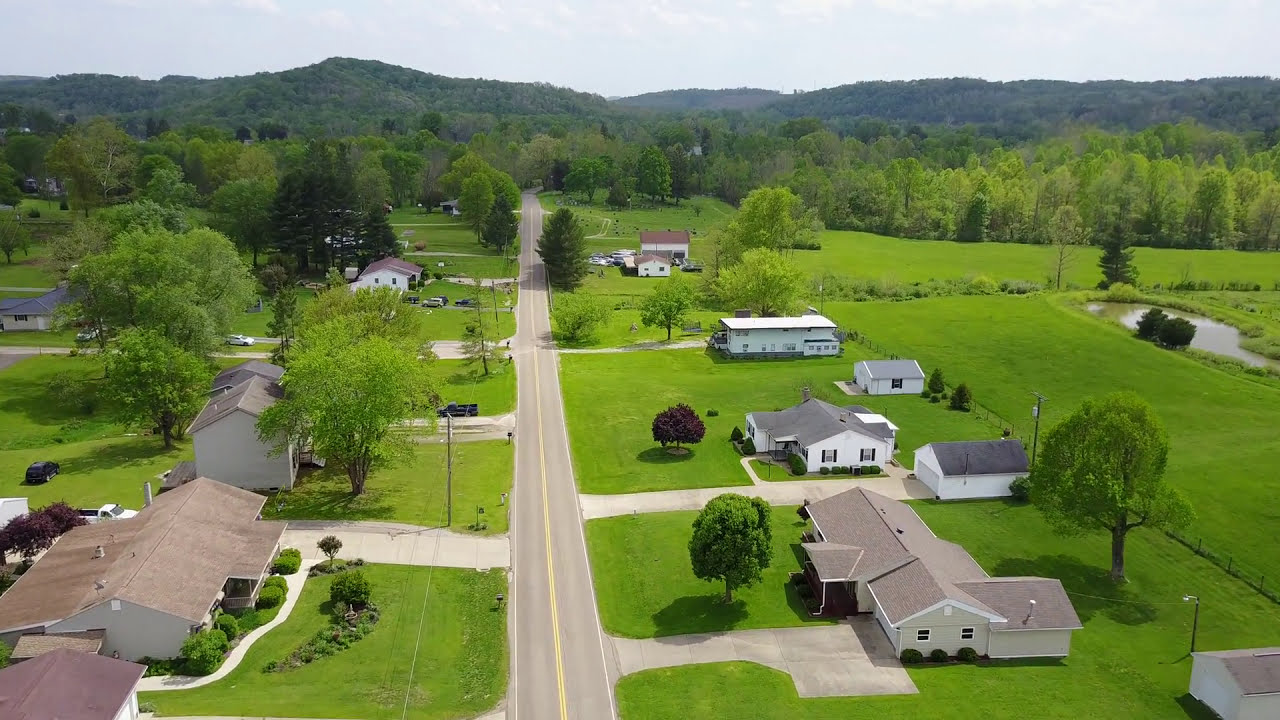This is a detailed aerial landscape photograph depicting a serene, rural subdivision, possibly in the Midwest. The center of the image features a straight, two-lane paved road, distinctly marked by double yellow lines, running from the bottom towards the top. Flanking the road on both sides are spacious, tidy ranch-style homes, most with lush, green lawns and some detached garages. Notably, a large home with a red roof and front landscaping stands to the left of the road in the foreground, neighboring another house surrounded by tall trees, with a third house visible farther down. On the right side, a single-story beige house with a brown roof and a prominent tree in the backyard faces a green pasture area, accompanied by a white house with a detached garage and more residences extending down the street. The clear sky above, dotted with clouds, frames a dense forest and distant green mountains, adding depth and a natural backdrop to the idyllic, middle-class suburban scene captured by a drone in the middle of the day. The color palette includes shades of green, gray, yellow, brown, red, maroon, white, and purple, emphasizing the tranquil, picturesque setting.